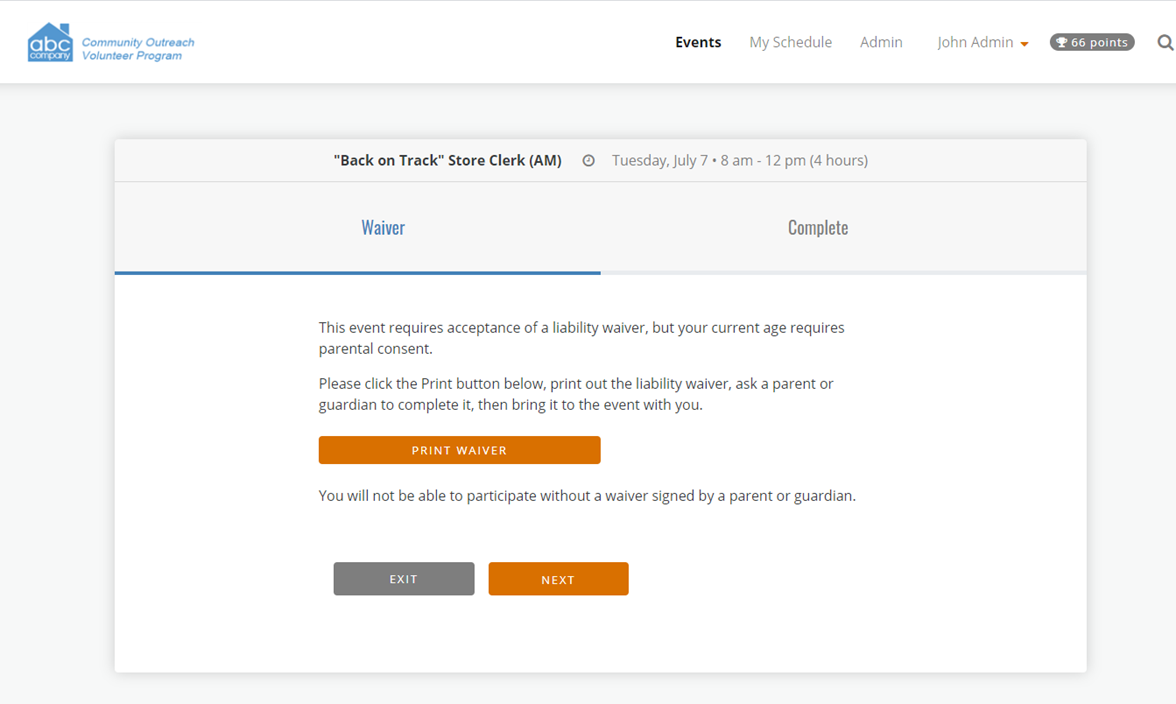**ABC Company Community Outreach Volunteer Program – Event Details Screen**

The screenshot depicts a web interface for the ABC Company Community Outreach Volunteer Program. At the top of the screen, there's a white menu bar featuring tabs labeled "Events," "My Schedule," and "Admin." The username "John admin" appears alongside an orange downward-facing triangle icon, suggesting a dropdown menu. 

A trophy icon adjacent to the text "66 points" is enclosed within a gray capsule shape. To the right of this is a search option. A subtle shadow underlines the menu bar, enhancing its contrast against the white background of the interface. Below, the main content area consists of a pop-up window.

The pop-up window details an event: 
- Title: "Back on Track, Store Clerk AM"
- Date: "Tuesday, July 7th"
- Time: "8 AM to 12 PM" (totaling four hours)
  
The window contains options labeled "Waiver" (highlighted in blue) and "Complete," with a blue line indicating the selected option. Below this line, a message indicates the event requires the acceptance of a liability waiver and mentions parental consent due to the participant’s age.

Detailed instructions follow:
1. Click the "Print Waiver" button to print the liability waiver.
2. Have a parent or guardian complete the form.
3. Bring the signed waiver to the event.

A large, wide, orange button labeled "Print Waiver" is prominently placed for user action. Beneath this, a cautionary note emphasizes that participation cannot proceed without the signed waiver. Finally, two action buttons are available at the bottom: a gray "Exit" button on the left and an orange "Next" button on the right.